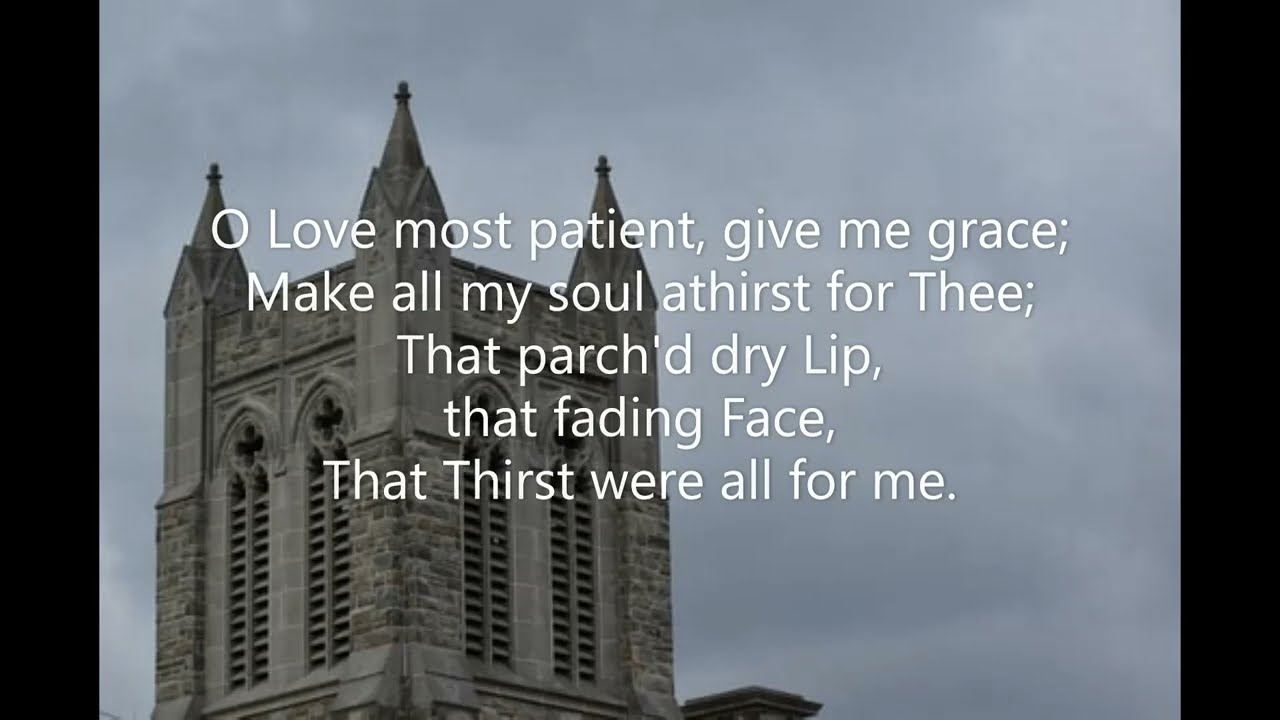The image features a striking church steeple set against a bluish-gray sky with black vertical stripes on the left and right borders. The stone church, predominantly gray with hints of darker shading, occupies much of the left side of the picture, showcasing the top of the steeple. The steeple has three pyramid-like cones, each crowned with crosses, giving the structure a distinctive silhouette. There are also four arch-like vents resembling windows—two on each side—with clover-shaped openings above them. These elements suggest the possibility of a bell within the steeple. Superimposed on the image in white font, the text reads: “Oh love most patient, give me grace, make all my soul a thirst for thee. That parched dry lip, that fading face, that thirst were all for me.”